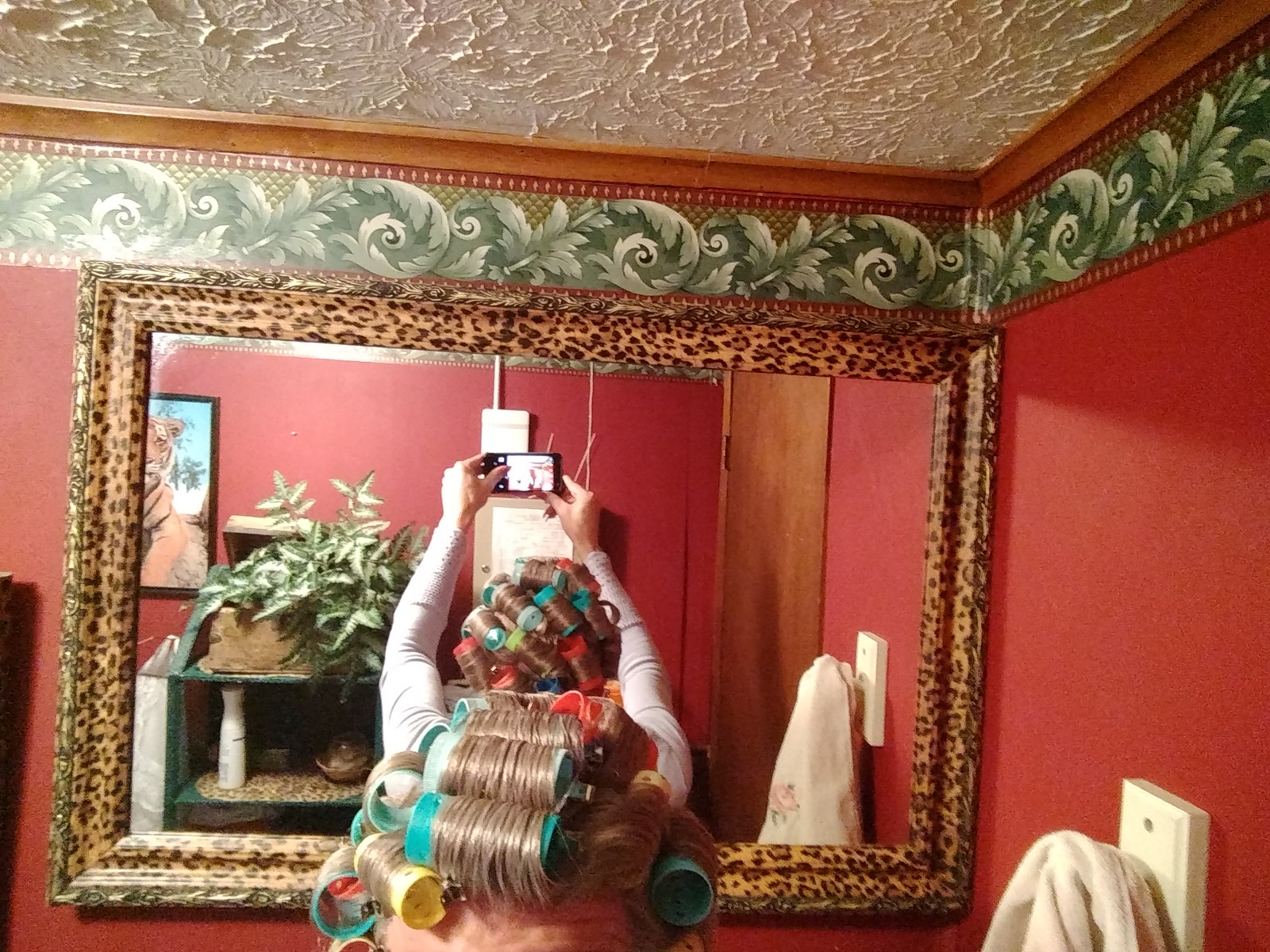In this vibrant photograph, a person is awkwardly taking a selfie in a red room, using a large leopard-print framed mirror to capture the back of their head adorned with large, multicolored hair curlers, including red, green, and yellow ones. The individual is wearing a long-sleeve pink top and has blonde hair. Their arms are extended upward, holding their phone overhead to snap the picture. The room features walls painted in a richly saturated dark red, with a green floral-patterned border running near the stucco-textured ceiling, which has brown trimming. Additionally, a towel hangs on a rack to the right, adding to the detailed setting of this unique scene.